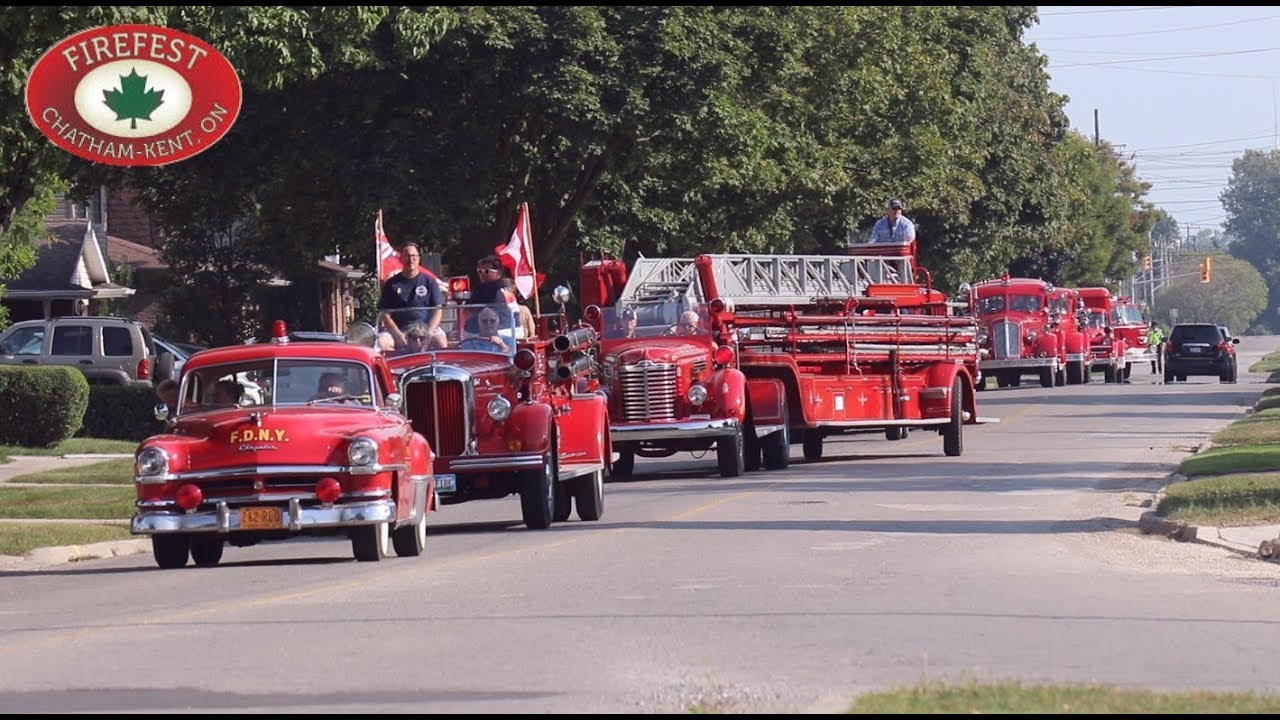The image captures a vibrant scene at Firefest in Chatham-Kent, Ontario, showcasing a parade of vintage firefighter trucks. On the left, an oval red sign prominently displays "Firefest, Chatham-Kent, ON" with a green maple leaf. The procession begins with a classic red FDNY sedan, boasting a bubbly design and yellow-accented Chevrolet details, followed by a series of old-fashioned fire engines, including a convertible truck with a ladder. The street is lined with lush green trees arching over the scene, while beige, tan, and white houses with various roof colors—black, brown—peek through the foliage. The roadway itself is a smooth gray surface punctuated by yellow traffic lights, grassy curbs, and additional vintage fire trucks stretching into the distance. On the right side, beside more fire trucks and a black SUV, a person in yellow and black stands in the street, possibly conducting traffic. The overall colors present in the image are vibrant reds, grays, beiges, tans, greens, blacks, blues, yellows, and lime green, framing a nostalgic glimpse into this elaborate display of fire service history.